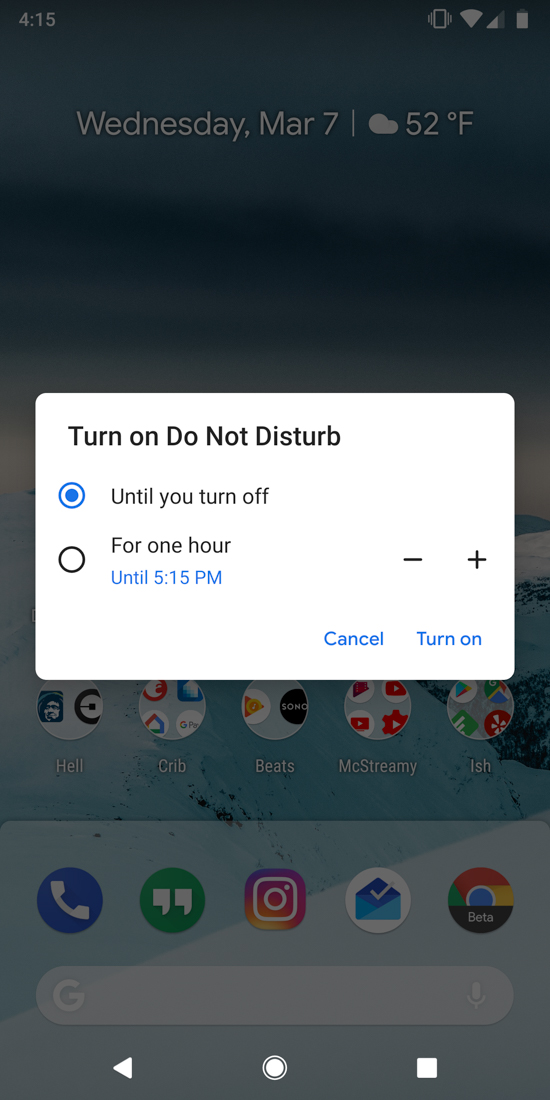The image appears to be a screenshot of a smartphone homepage. In the top left corner, the clock displays "4:15." On the right side, there are several icons: a possible silence mode icon, a Wi-Fi icon, a signal strength indicator, and a battery life icon. Centered below these icons, the date is displayed as "Wednesday, March 7th," followed by a vertical line. Next to this, there is a cloud symbol indicating the weather, with "52°F" written beside it.

Overlaid in the center of the screen is a white rectangle with a black text header reading "Turn on Do Not Disturb." There are two selectable options: the top option, which is currently checked, says "Until you turn off," and the bottom option says "For one hour." There is also the text "Until 5:15" in blue, suggesting a clickable link to change the duration. To the right of this text, there are plus and minus signs for adjusting the time. At the bottom right corner of the white rectangle, there are two clickable links labeled "Cancel" and "Turn on."

Beneath this, five application folders are visible, arranged from left to right and labeled "Hell," "Crib," "Beats," "McStreamy," and "Ish." Below these folders, there are icons for a phone app, messaging app, Instagram, email, and some sort of Google beta app.